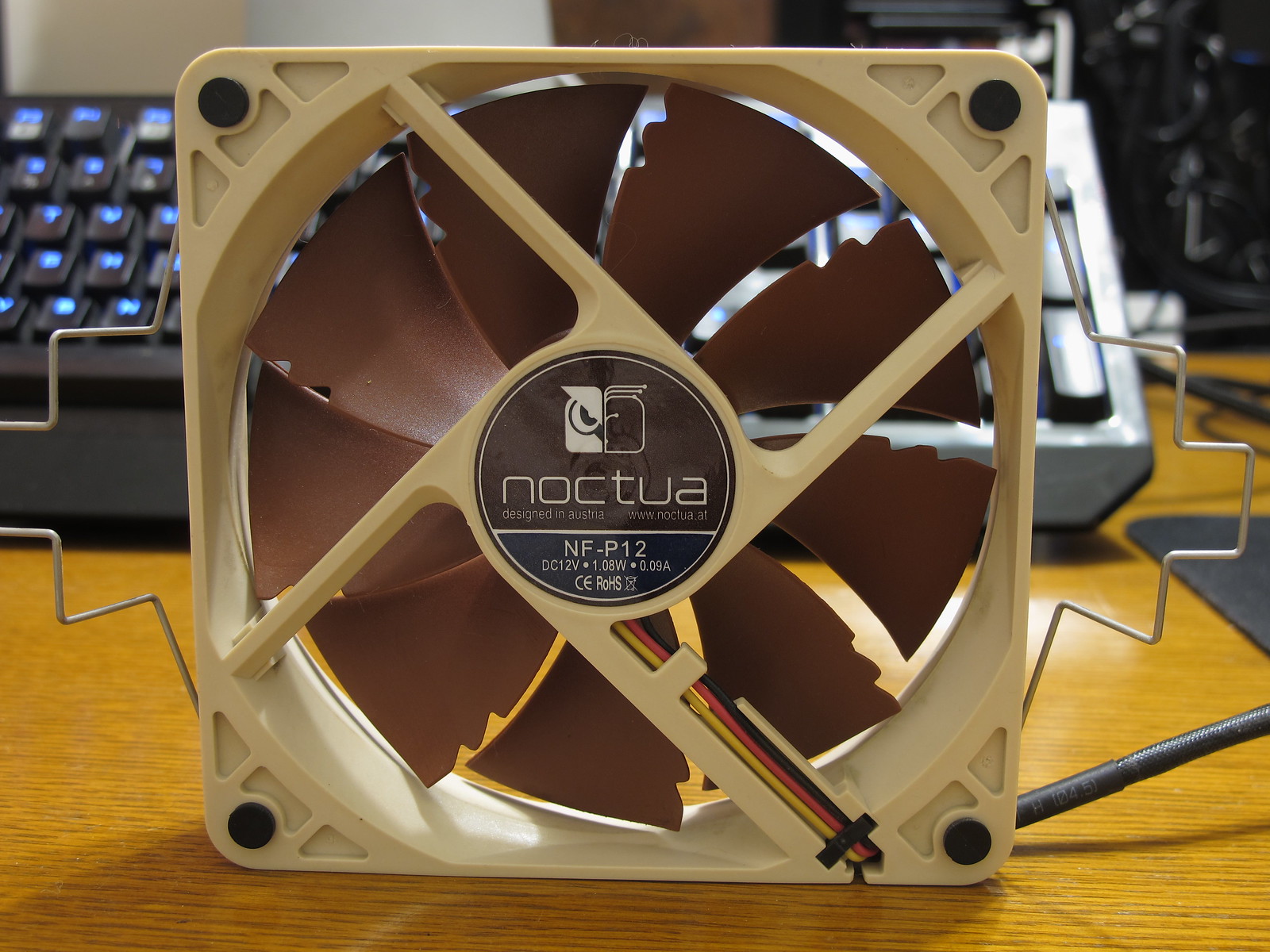This color photograph features a small computer fan prominently positioned on a brown, maple-colored desk, with a black keyboard illuminated by blue-backlit keys visible in the background. The fan, which likely belongs to a desktop computer's CPU unit, has a beige frame and brown blades, some of which exhibit jagged edges. Central to the fan is a circular sticker bearing the brand name "Noctua," written in lowercase letters (N-O-C-T-U-A) alongside an owl logo. The fan model is identified as NF-P12, with technical specifications indicating it operates at DC 12 volts and 1.08 watts. Electrical cords are attached to the right side of the fan, and the design is noted to have been crafted in Austria.